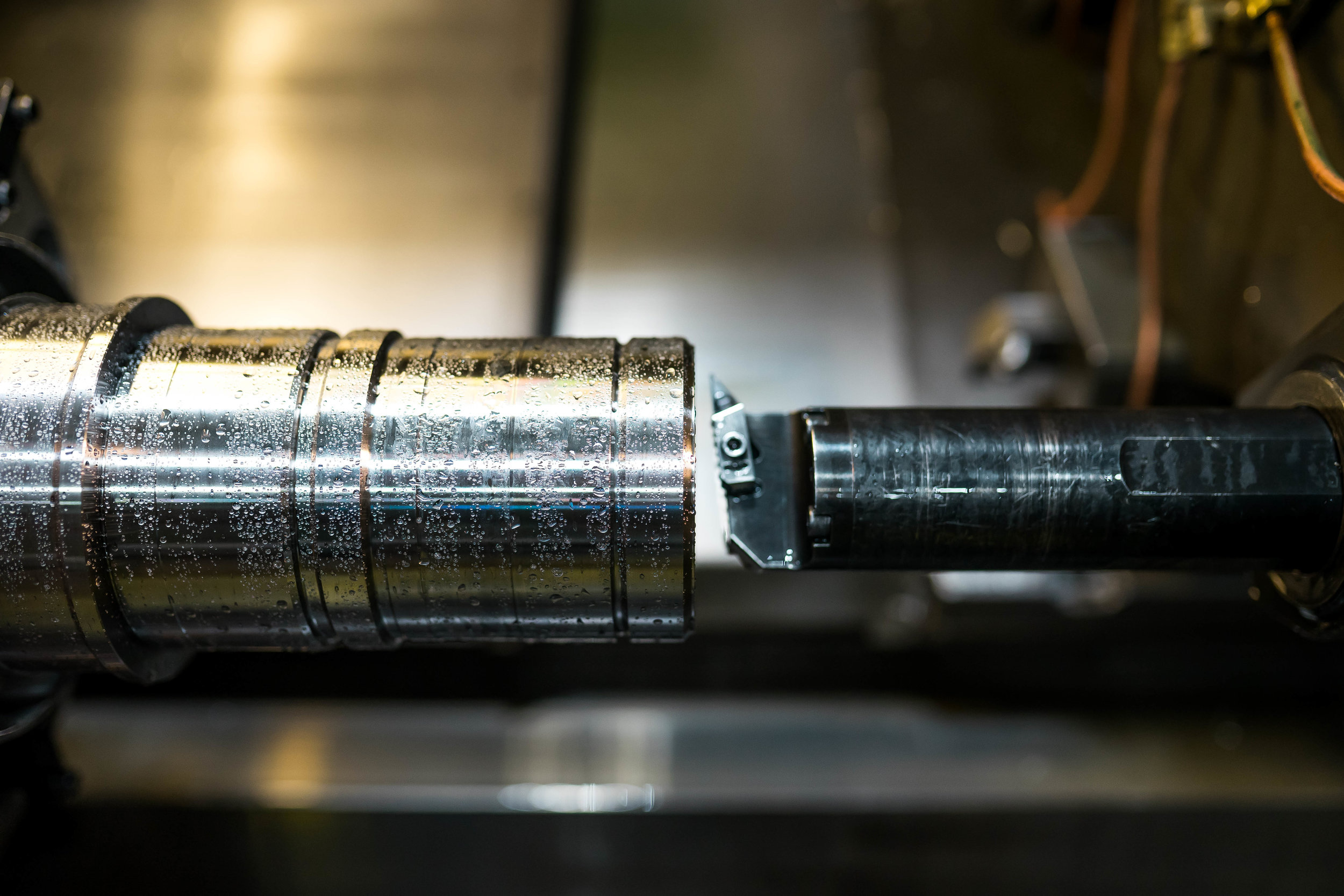The photograph captures a close-up view of two interconnected machine parts placed in what appears to be an indoor workshop setting. In the foreground, a smaller, black, cylindrical pipe with a rough, scratched surface emerges from the left, connecting to a larger, glistening, chrome or steel-like cylindrical object on the right that reflects light and appears almost glowing. This larger part, which is thicker at its base, gives off a golden-copperish hue, possibly due to lighting or reflections. Small water droplets or frost might be visible on the shiny surface, adding to its reflective quality. The two components are slightly elevated off a flat surface, with a gap between the bottom of the cylinders and the surface, connected by a flat, undefined shape. In the blurred background, other indistinguishable machine parts emphasize the primary focus on the contrasting and intricate details of the two main metallic components.